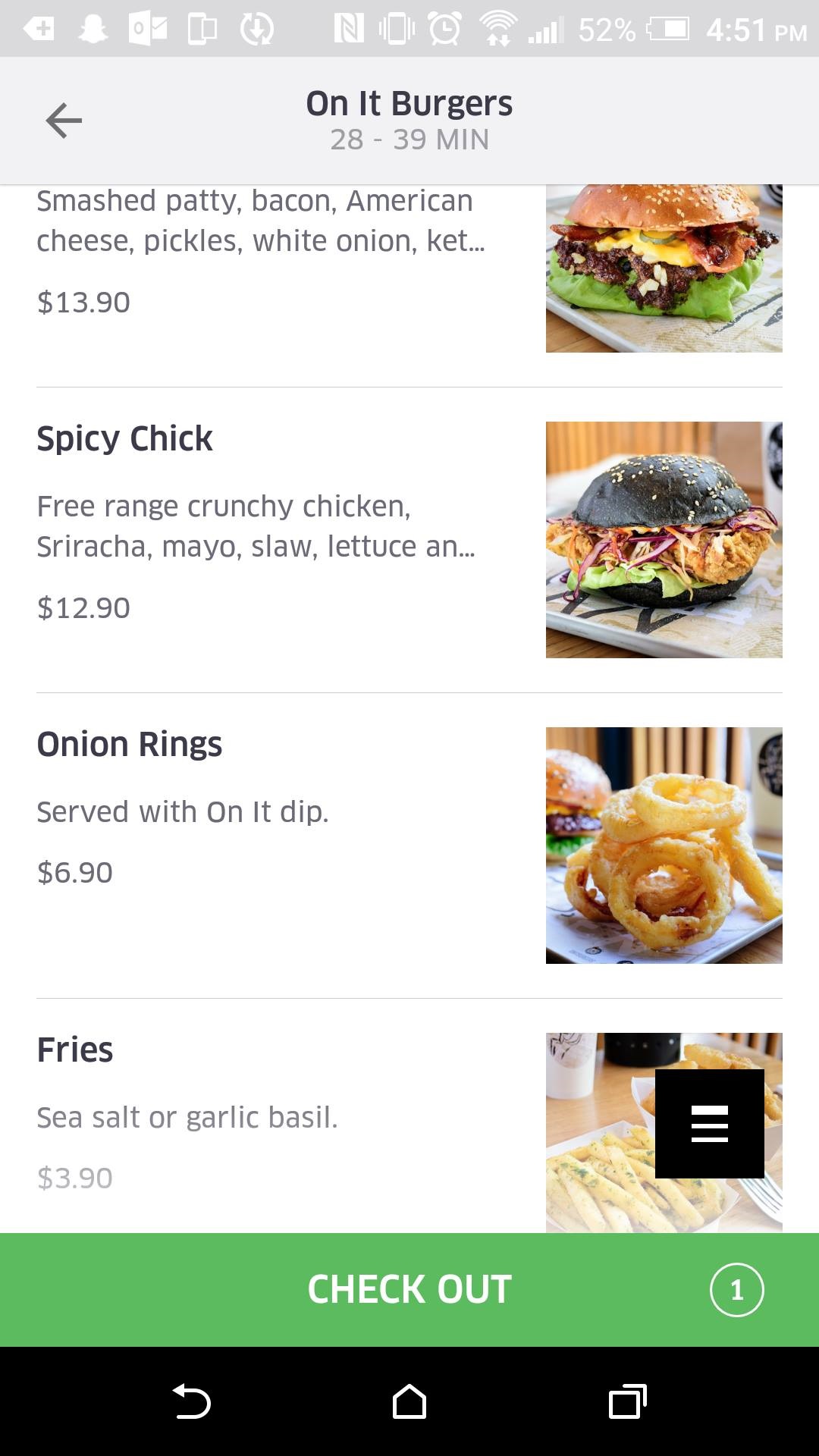The image showcases an Android phone displaying a food delivery app in the order summary screen. The phone features the signature back, home, and overview buttons at the bottom. Dominating the lower part of the screen is a prominent checkout button indicating one item in the cart and an estimated delivery time of 28 to 39 minutes.

The app displays detailed menu items, including:
- A "Smash Burger" priced at $13.90, which includes a hamburger with smash patty, bacon, American cheese, pickles, white onion, and ketchup.
- The "Spicy Chick" burger, featuring free-range crunchy chicken, sriracha mayo, slaw, and lettuce, priced at $12.90.
- Onion rings served with dip, costing $6.90.
- Fries seasoned with either sea salt or garlic basil, available for $3.90.

The status bar at the top of the phone's screen reads 4:51 p.m., showing a battery level of 52%, indicating an active cellular connection, alarm, Vibrate mode, and Wi-Fi connection. Icons reveal that Snapchat and Microsoft Outlook are running in the background among various other apps. The taskbar is densely populated with notifications and settings indicators, highlighting the user’s multitasking activity.